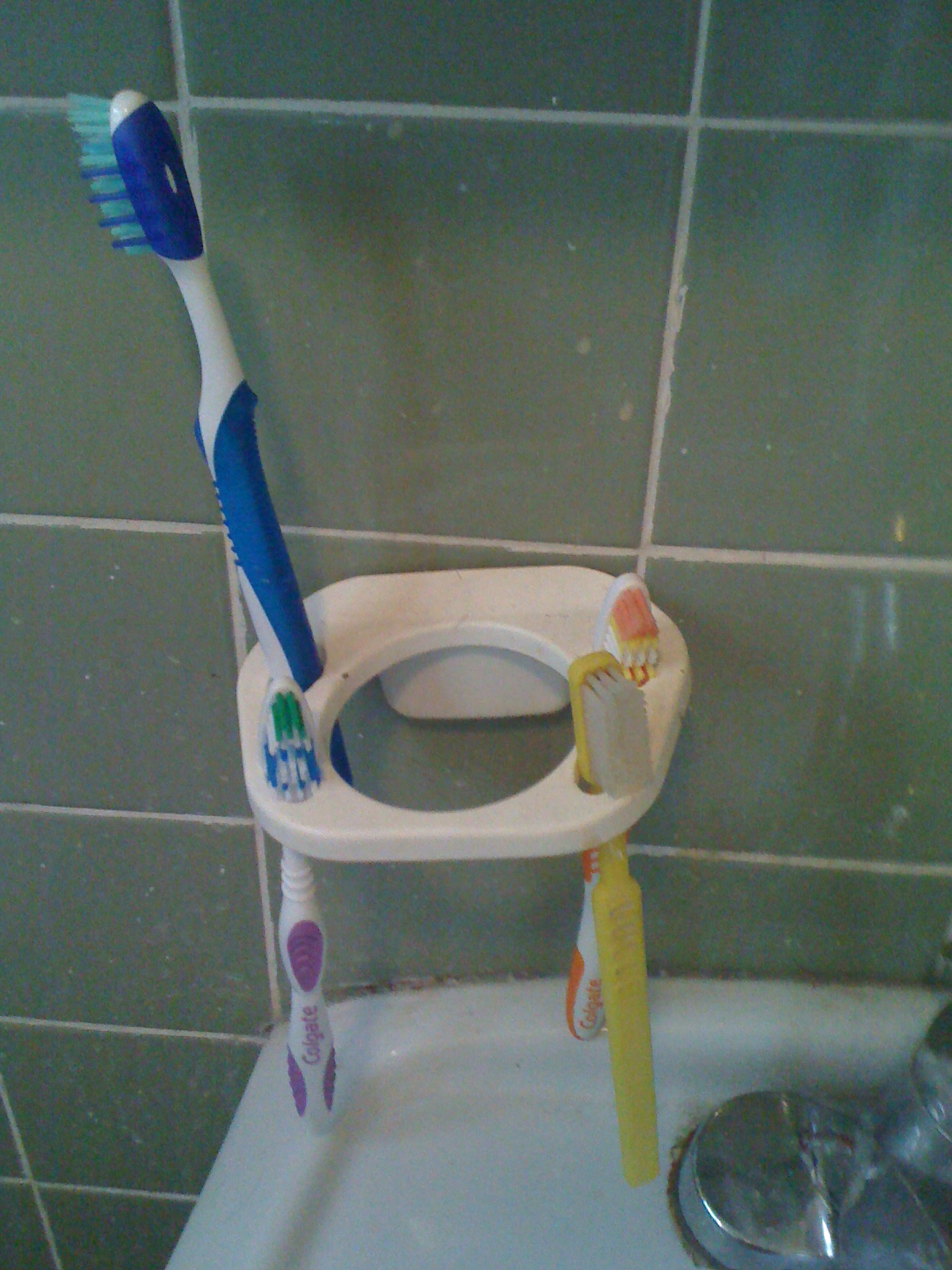The image depicts a small section of a bathroom featuring a wall with glossy, seafoam green tiles accented by white grout. In the lower right corner of the image, part of a sleek, white porcelain sink and a chrome faucet are visible, though the area around the faucet is marred by rust and toothpaste spatter. Mounted on the wall is a powder-coated white metal toothbrush holder designed to hold a tumbler in its central circular opening, though currently, it holds four toothbrushes in the surrounding slots. 

The toothbrushes are as follows: a tall blue and white toothbrush that doesn't fit neatly into its slot and thus protrudes above the others; a Colgate toothbrush in white with purple grips, featuring a double-textured head with circular and longer bristles; a simple yellow toothbrush with a yellow handle and head; and another Colgate toothbrush in orange and white. The holder appears quite grimy, adding to the overall impression of a well-used but neglected bathroom.